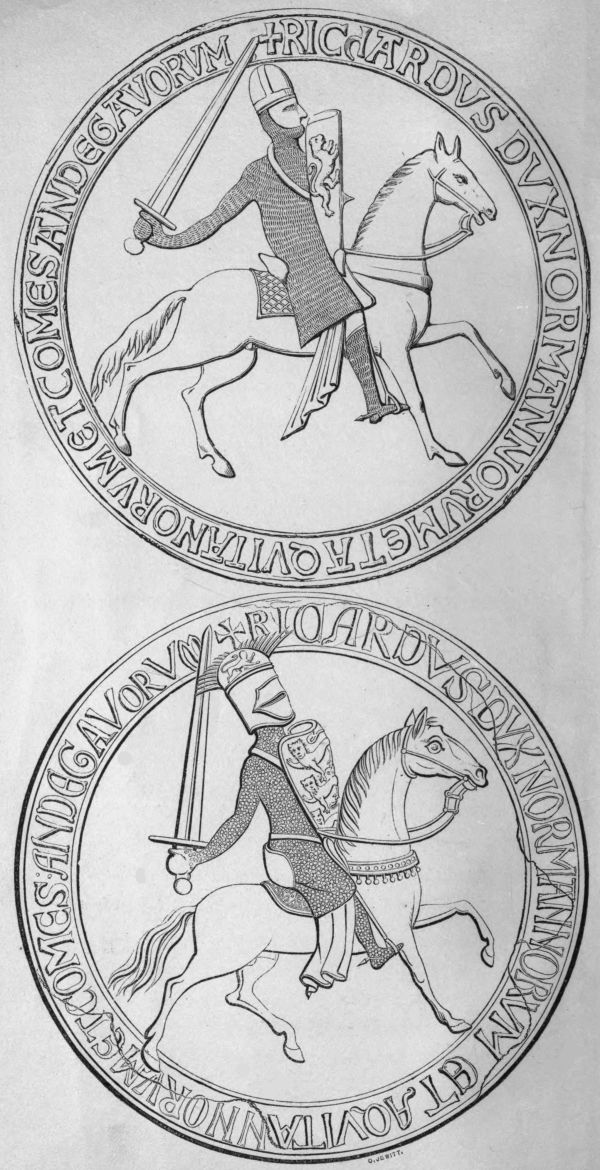The image showcases two circular coins featuring detailed illustrations of knights on horseback. In the top coin, a knight in full armor is depicted riding a horse, with his sword drawn high and a shield firmly gripped. Notably, his face is visible, lacking a helmet, and there is Latin script encircling the coin's edge. The bottom coin presents a similar yet distinct image: a knight, also in full armor, with his sword raised in a slightly more upright position and a shield held against his chest. This knight wears a helmet, obscuring his face. The horse in the bottom coin is depicted with more luxurious features, including flowing hair and wide-open eyes. Latin inscriptions also border this coin, adding to its intricate design.